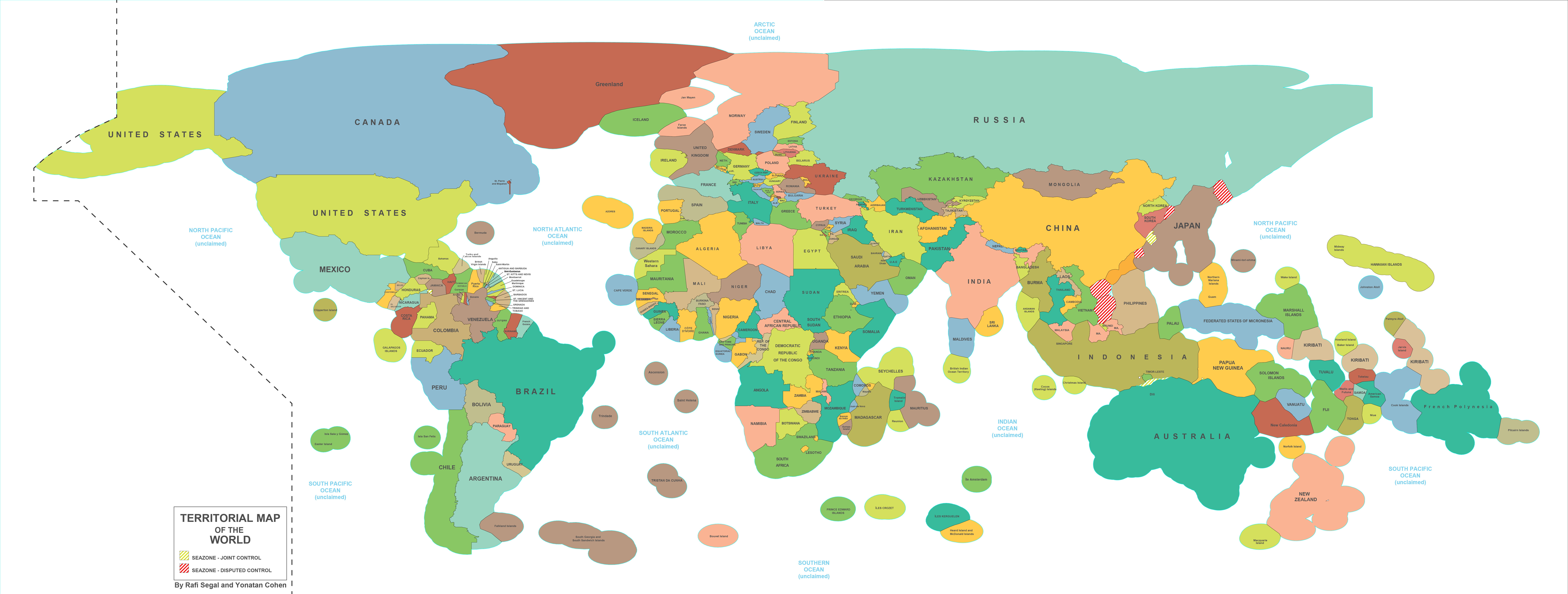This image depicts a detailed territorial map of the world set against a white background. At the bottom of the map, there is a small box containing a legend and the title "Territorial Map of the World" in black text. The legend includes color swatches such as light green and peach, but the accompanying text is too small to read clearly.

The United States is prominently shown in green, situated below Canada, which is colored blue. Adjacent to the mainland United States on the left, Alaska and Hawaii are also notable. Mexico, along with various smaller islands, is visible below the United States. South America is mapped out with countries like Brazil and Colombia clearly marked.

The vast expanse of Russia is depicted in turquoise, dominating the map, with China below it in yellow. Europe comprises diverse colors—blue, peach, green, light green, lime green, and beige—highlighting its numerous countries. Australia is colored green, accompanied by smaller surrounding islands.

Overall, the map provides a color-coded representation of the world's continents and countries, though the text labeling the countries is quite tiny and difficult to read.